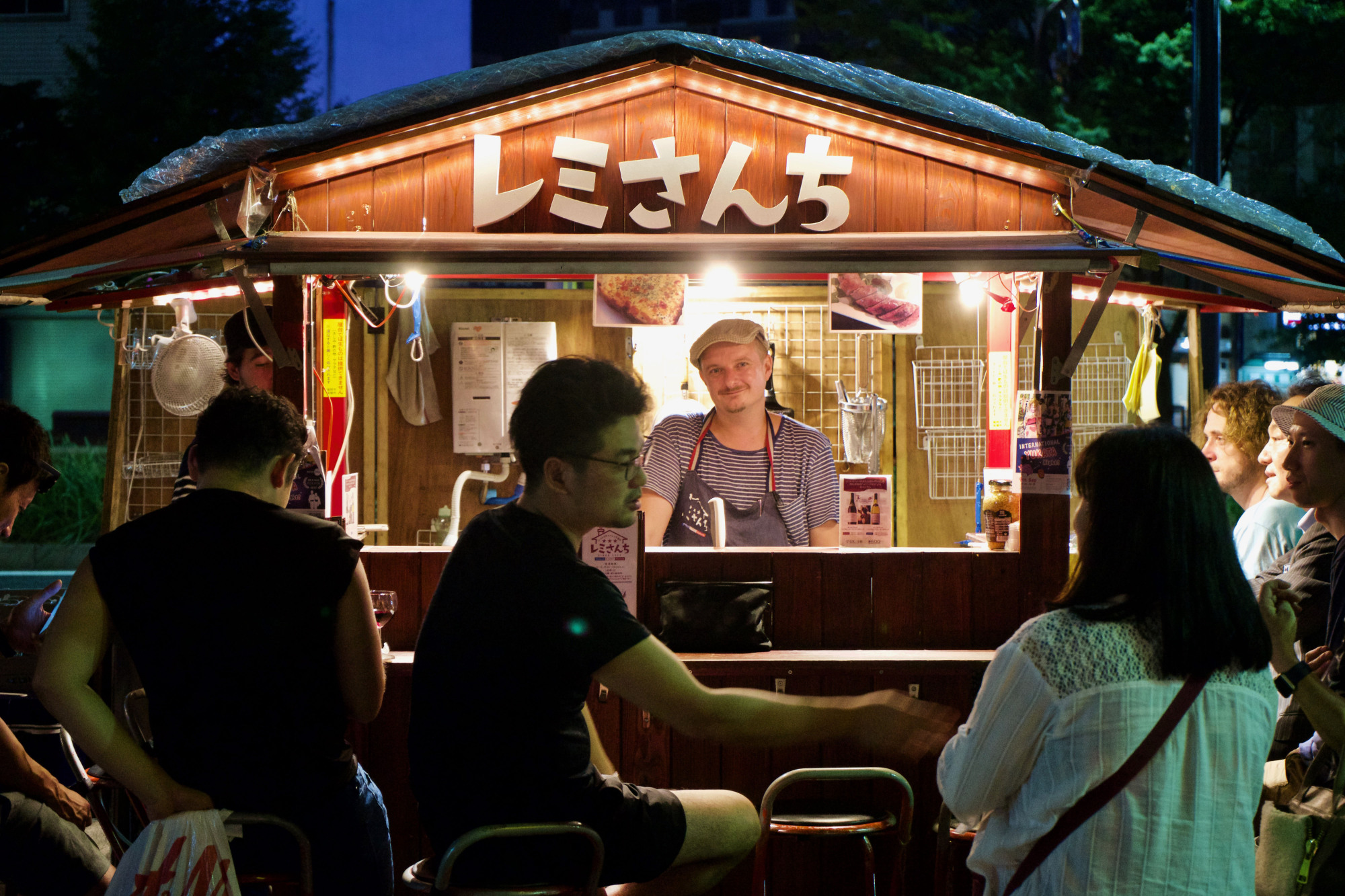This photograph captures a delightful outdoor tiki hut bar styled as a small restaurant. The Caucasian bartender, with strawberry blonde hair and a slight smile, is positioned at the center of the scene. He is wearing a navy blue apron with red, white, and blue strings over a short-sleeved, light and dark gray striped t-shirt, along with a cap. The overhead triangular roof is wooden, and beneath it, the name of the bar is displayed in white Cyrillic letters, although some perceive them as Japanese symbols spelling "L-E-J-H-5". Inside the hut, the background features menu pictures depicting hot dogs and pizza, along with racks on the wall.

In front of the bartender is a small countertop where six young patrons are seated, engaging in various activities such as chatting, checking their phones, and interacting with one another. The front bar area also has additional seating on the side. The setting is lush with trees and a blue sky in the background. The female patrons include one wearing a white blouse with long black hair, another sporting a green cap, and a third with a long hair conversing with a man. The males are dressed in casual attire, with one notably wearing blue shorts and a dark shirt. Above the bar, a plastic wrap is bunched up on the ceiling, adding to the quaint and makeshift aesthetic of the food stall. The overall atmosphere is casual and inviting, set amidst a picturesque outdoor environment.